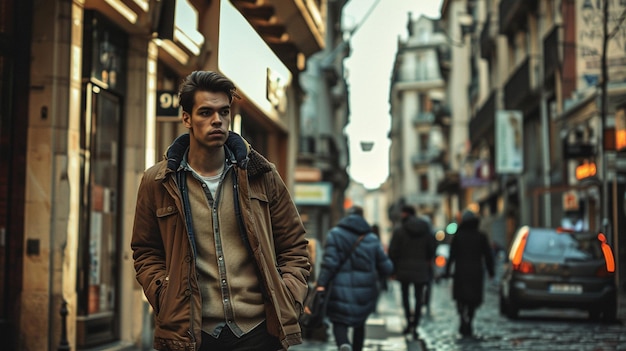In this photograph, a young man, approximately 30 years old, stands prominently in the foreground, slightly off-center. He is dressed warmly in a thick brown coat layered over a sweater and a shirt. His hair, not quite short but neatly combed back with product, adds a touch of sophistication to his appearance. The backdrop reveals a narrow, European-style street lined with quaint shops. A small car is parked further down the street, and several pedestrians, walking in the opposite direction, are captured out of focus, adding a dynamic yet serene ambiance to the scene. The overall composition emphasizes the man's presence while offering a glimpse into the everyday life of the charming locale.